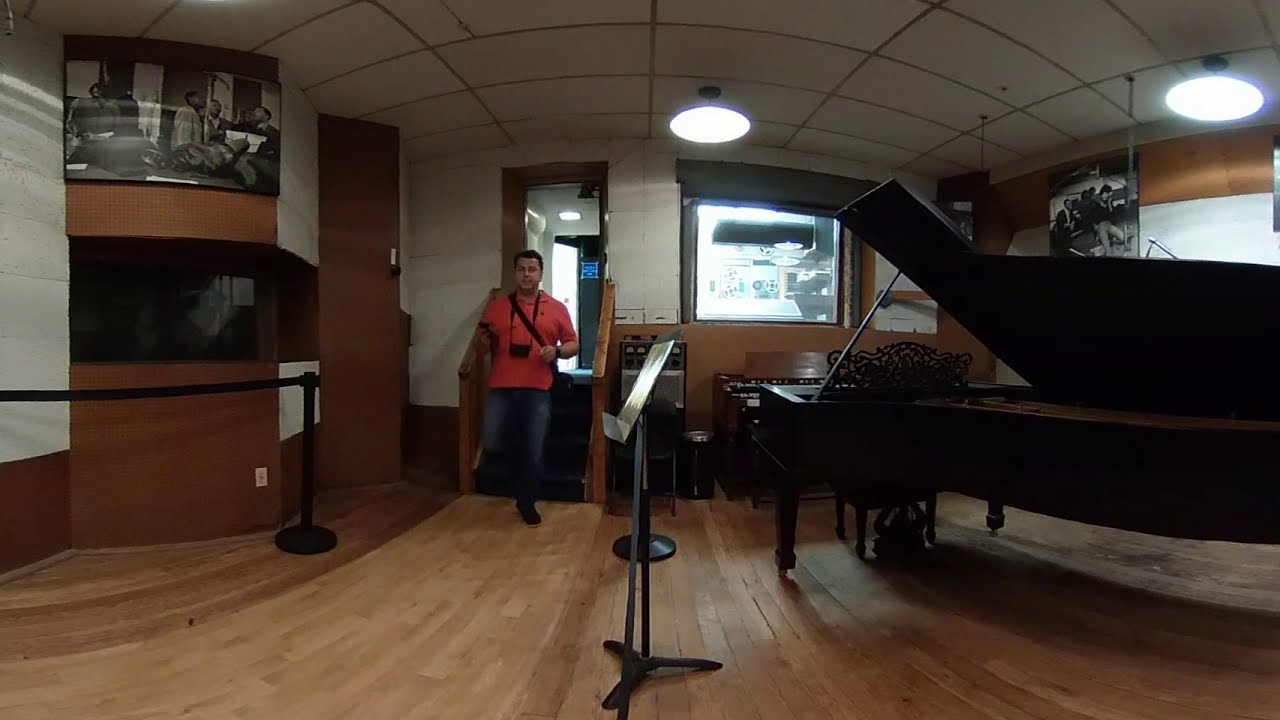In the detailed scene of a music studio, a man wearing an orange shirt and blue jeans is walking through a doorway. He has a black cross-body strap, possibly for a camera, visible against the white ceiling and hardwood floor. The studio contains a variety of musical elements: notably a grand piano with its lid open on the right side of the image, and a black music stand positioned centrally in the room. The ceiling hosts two round lights, one in the middle and the other towards the upper right corner.

Adjacent to the man’s entry point are amplifiers and a large window, likely indicating a recording area behind him, which is brightly lit compared to the dimmer foreground. On the upper left wall, there’s a framed picture of African American musical artists. Directly below the picture are black stanchions, resembling queuing barriers one might find in a theater. In the lower left quadrant, there is a black barrier, which adds to the organized layout of the studio.

Subtle details suggest the image was captured with a 360 or wide-angle lens, as indicated by the distortion, particularly in the ceiling. Finally, in the left-hand side of the image, mounted on a shelf, appear two stacked TVs, adding to the room’s eclectic mix of equipment and decor.